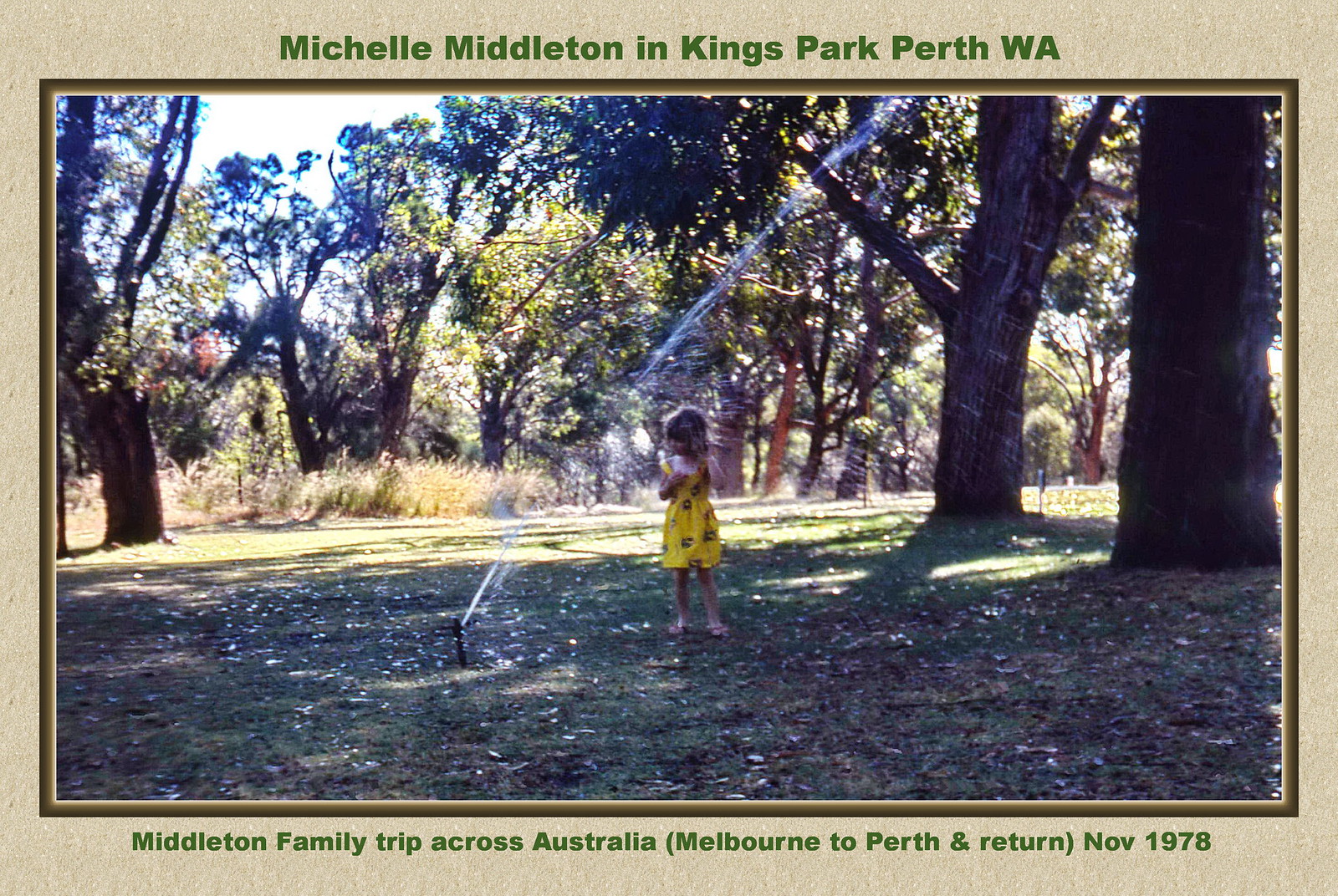This photograph, taken during the Middleton family's trip across Australia from Melbourne to Perth and return in November 1978, captures a joyful moment in Kings Park, Perth, WA. The image features a young Caucasian girl named Michelle Middleton, with short blonde hair, wearing a patterned yellow dress. She is playing near a water sprinkler that sprays up towards the sky. The scene is set on a sunny day with a clear blue sky, featuring lush green grass and numerous leafy trees, including two prominent ones behind her—one with a thick trunk and another with abundant branches. The natural setting includes additional brown tree trunks and scattered dead leaves on the ground, creating a picturesque backdrop. The image is framed with a Manila border, and green text at the top reads "Michelle Middleton in Kings Park, Perth, WA," while the bottom text states "Middleton family trip across Australia, Melbourne to Perth and return, November 1978."